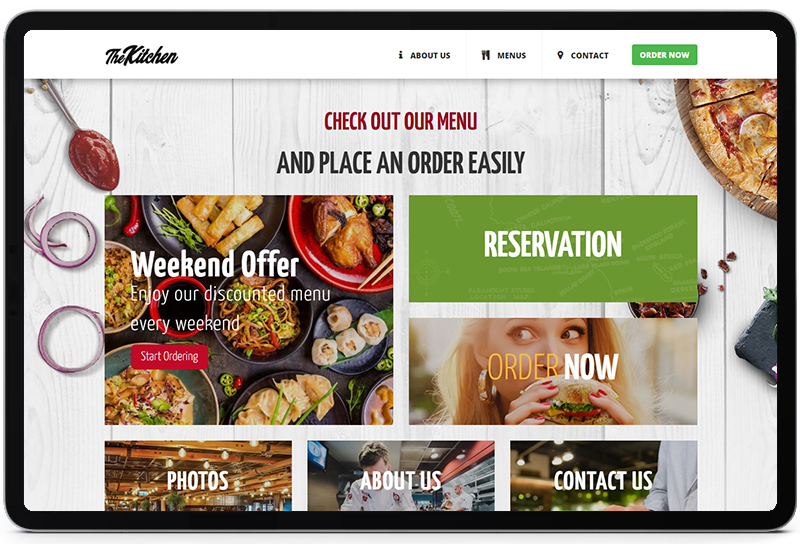This image features a user interface with a black-edged design. In the top left corner, a navigation menu includes options labeled "The Kitchen," "About Us," "Menus," "Contact," "Order Now," and "Table." Below the menu, there is an image of a spoon with red ketchup and red onions, accompanied by a prompt to "Check out our menu." The interface then encourages users, "You can place your order pretty easily," and shows an appetizing pizza with the question, "What should I choose?"

In the top right corner, additional menu options are displayed, including "Reservation," "Order Now," and "Bonus Content." Below that, labels for "Photos" and another repeating "Photos" section are visible. The scene includes a depiction of a person in a room with wooden bins. Another element in the top left announces a weekend offer: "Enjoy our discounted menu for the weekend, start ordering."

The visual content further showcases bowls of noodles, chicken, egg rolls, and dumplings to entice customers. In the top right, the word "Season" appears. The table featured in the center of the image is described as white with some green hues, and it appears to be divided into boards.